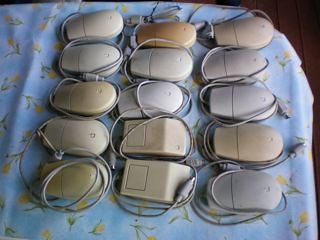The image depicts a collection of 15 vintage computer mice meticulously arranged in a three by five grid on a surface covered with a white sheet adorned with yellow floral designs. Most of the mice are the typical rounded shape, with a beige color indicating heavy use over time, while a few in the middle of the bottom row are distinctly squared with a large square button on top. The cords of each mouse are neatly wrapped around their respective bodies. A brown wooden surface peeks into the frame in the upper right corner, adding a touch of contrast to the detailed display of retro tech against the floral sheet.